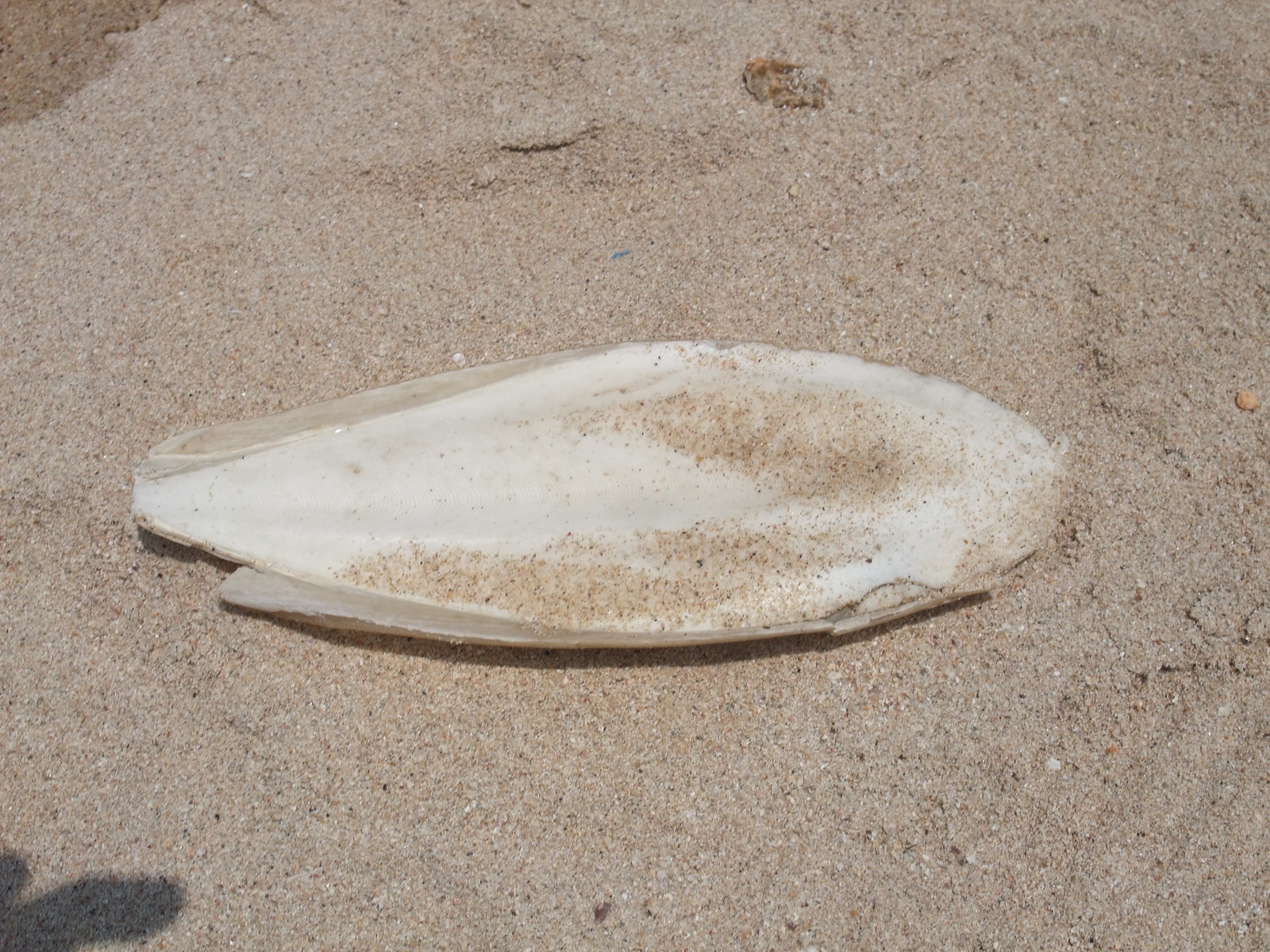The photograph depicts a teardrop-shaped white object, possibly a shell or sea creature, partially embedded in clear, golden, speckled sand. The tip of the teardrop points to the left while the rounded end faces the right. Gray ridges are visible on its sides near the teardrop's point. The white object's smooth, opaque surface is dusted with tan and brown sand particles. It sits centered both horizontally and vertically within the frame, set in an outdoor, sandy environment on a sunny day, inferred from the lighting. The gritty sand background is interspersed with small rocks and debris, and there is a small, black shadow in the bottom left corner of the image, with a wet patch visible in the surrounding sand. The camera angle is an overhead shot, capturing the object from above.